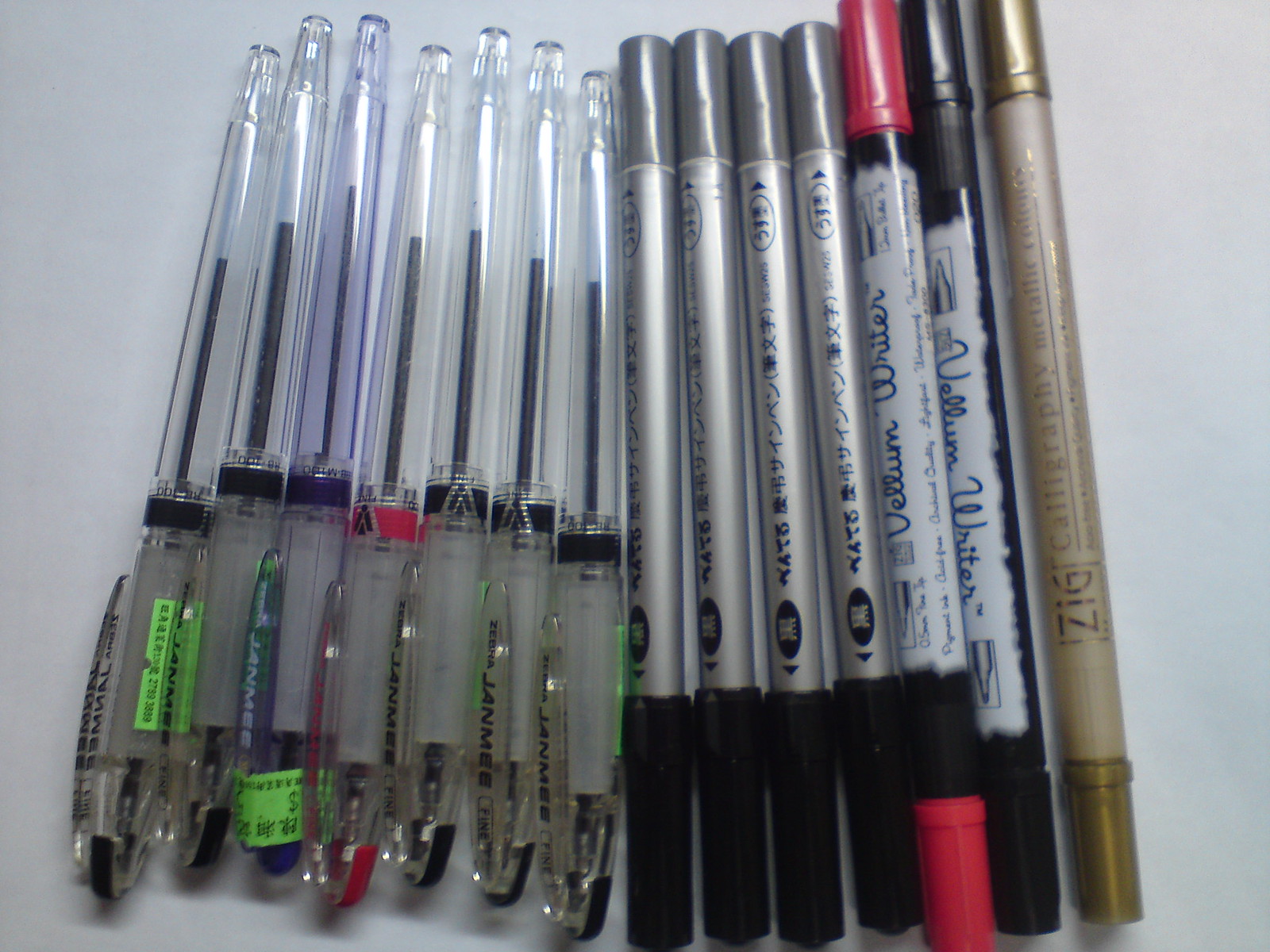This image displays an array of 13 pens laid out on a white surface. On the left side, there is a row of seven clear pens, each revealing the ink inside with color bands near the tip. These bands include black, purple, and hot pink colors. The clear caps complement the transparent bodies, while two of these pens have light green price tags attached. 

Immediately to the right are four pens with silver bodies adorned with what appears to be Chinese writing and finished with black caps. These pens have a more artistic look compared to the clear ones.

Next, there are two distinctive pens. One has hot pink caps on both ends and features a white body with black lettering, while the other one is primarily black with white writing and black caps on either end.

The final pen in the row is gold and marked with "calligraphy," suggesting its purpose. It also has gold caps on both ends, adding a luxurious touch to its appearance. The pens showcase a diverse range of designs and colors, making for a visually intriguing arrangement.